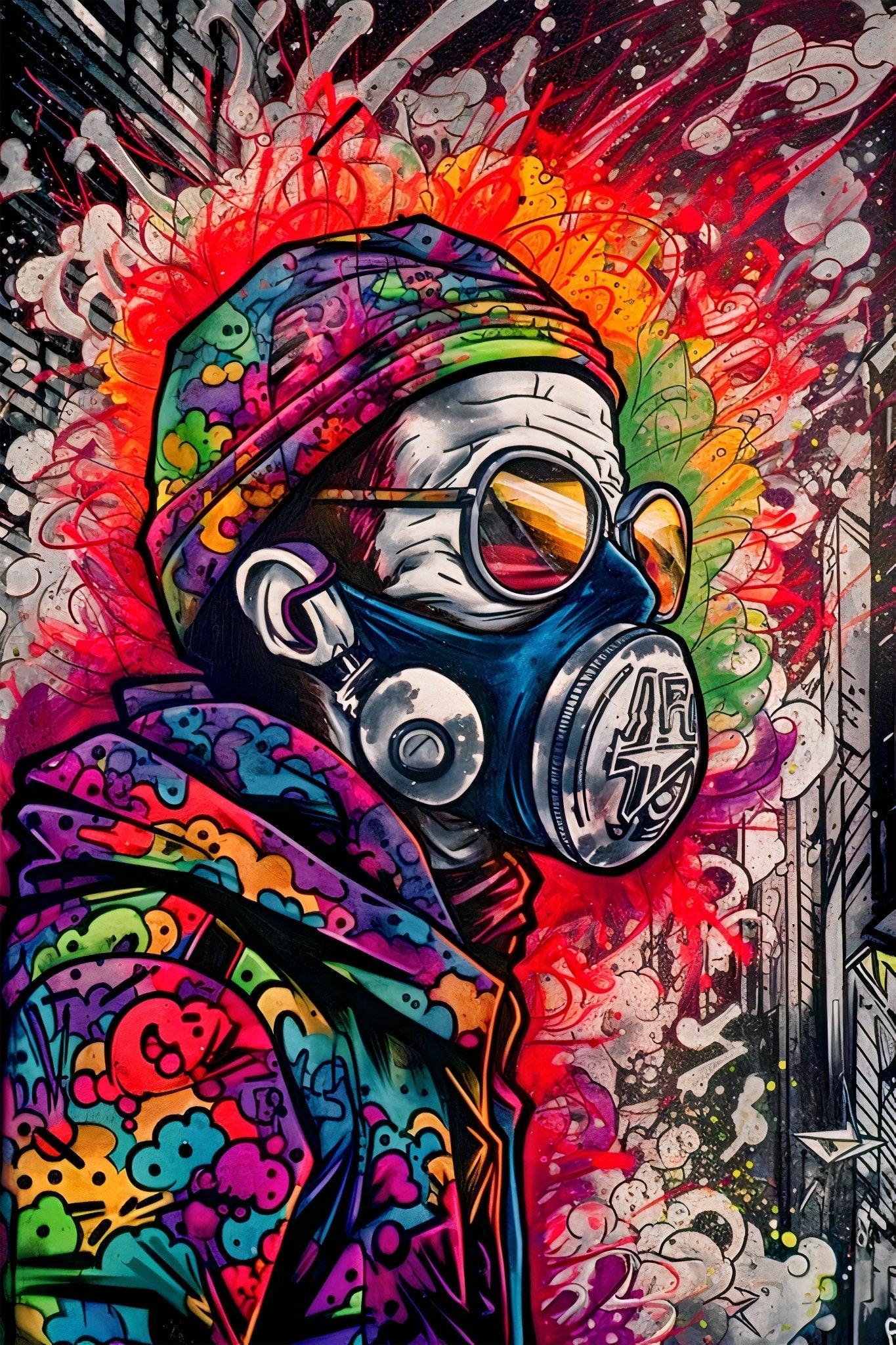The artwork features a vivid, graffiti-style poster of a graffiti artist in a long, vertical rectangular format. The artist is depicted in black and white, standing out against his colorful surroundings. He wears a bright, whimsical hoodie adorned with cute, silly round character faces and a matching knit skull cap. His face is obscured by aviator sunglasses and a blue painter's face mask with silver breathers. Surrounding the artist are plumes of vibrant, multicolored smoke in reds, oranges, blues, and greens, creating a striking halo effect. This colorful explosion contrasts sharply with the monochrome background, which showcases sketched images of tall skyscrapers. The base of the picture is predominantly black, adding depth to the dynamic scene. The entire composition invites the viewer to imagine the backstory behind the artist's enigmatic presence amidst the chaotic yet mesmerizing interplay of colors and elements.